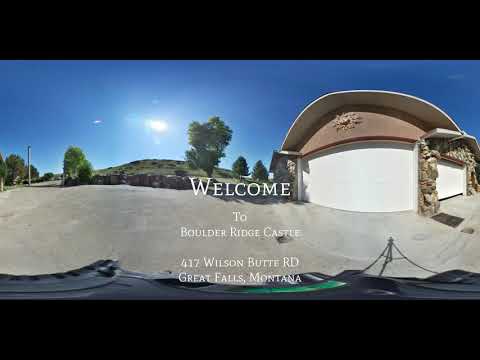The image depicts a daytime outdoor scene, most likely taken in a parking lot area. The upper part of the image shows a clear blue sky with the sun shining from the left-hand side, illuminating rolling hills and verdant green trees. Towards the right-hand side, there is a distinctive circular garage-like building featuring white walls and an elaborate stone archway. The building’s roof is characterized by a brownish top with a curved semicircular white canopy that extends over two white garage doors. The driveway beneath is a gray cement tarmac, complemented by a black surface stretched along the bottom border of the image, with the shadow of a tripod visible in the bottom right-hand corner.

In the very center of the image, there are five lines of white text that read: "Welcome to Boulder Ridge Castle, 417 Wilson Butte Road, Great Falls, Montana." The scenery includes a backdrop of green hills dotted with trees near their base, adding to the picturesque nature of the setting. The overall composition suggests a welcoming entrance to the mentioned location, highlighted by the sun and natural greenery.